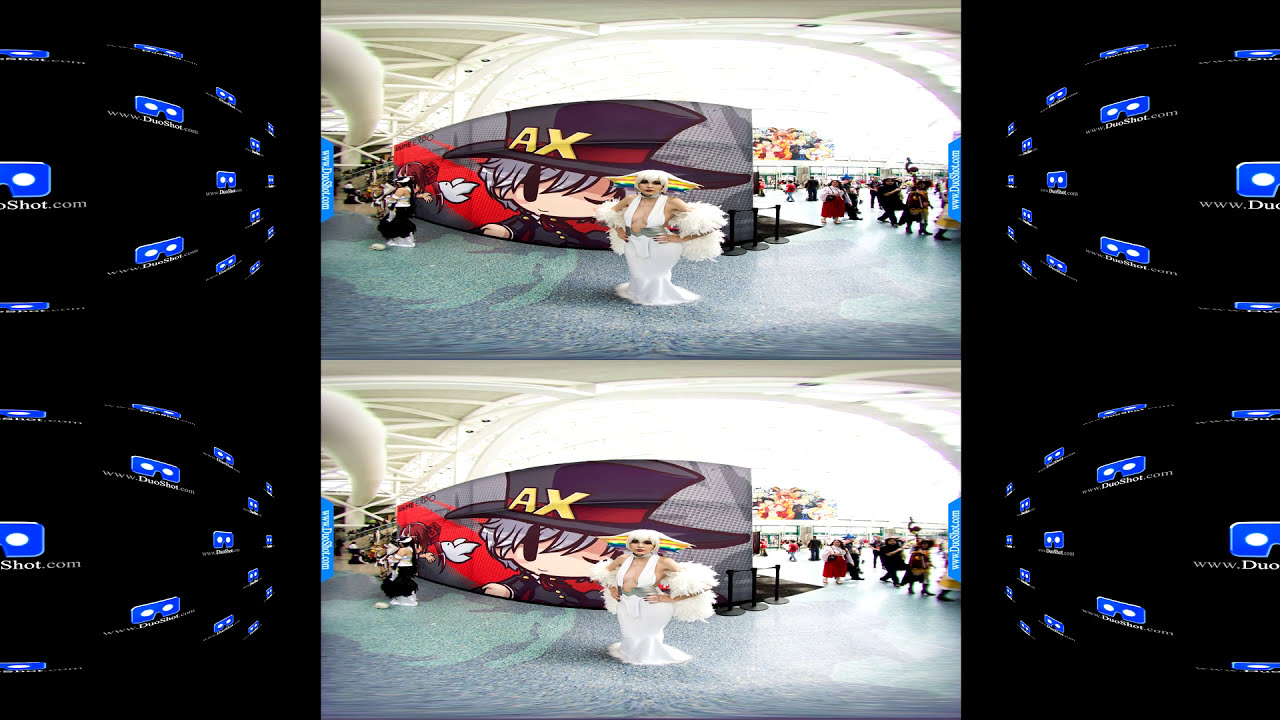The image consists of two almost identical frames, one on top of the other, both taken through a fisheye lens, causing significant distortion and warping the proportions. In the foreground, there's a woman in an intricate white dress that is sleeveless and features a bow wrapped around her arms and down her back. The dress reveals an open front down to her stomach and flares out slightly at the bottom. She is also wearing a large white hat. The background features a prominent banner with gray and black stripes on the right side, a purple section in the middle, and a red section below. The letters "A" and "X" in light gold color dominate the center of the banner, below which is an image of an anime character with gray hair and a blue shirt. Flanking the banner on both sides are rotating images of blue 3D glasses with white dots in the middle. Additionally, the sides of the image are bordered in black, featuring the text "duoshot.com" repeatedly. The backdrop includes a crowd of people and a bright white ceiling that grows more intense as it recedes. The ground is primarily blue with white speckles, transitioning to light green towards the left. The overall scene suggests a busy event or convention setting, possibly showcasing new products.